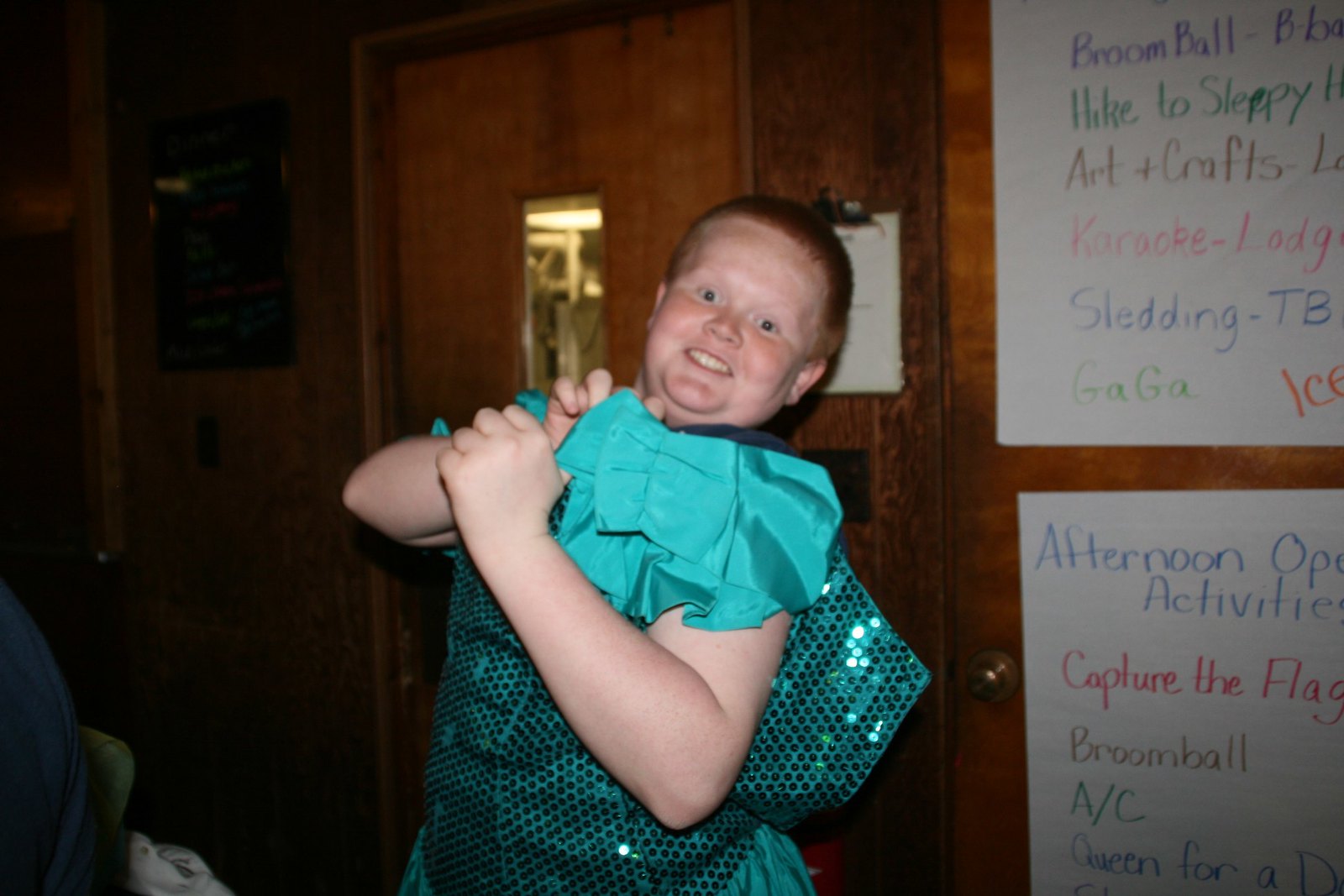The image showcases a young, white child, around 8 years old, with reddish, buzz-cut hair, wearing a vibrant, turquoise dress adorned with sequins. The dress, which has a high ruffled collar reaching up to the neck, creates an impression of playful confusion as the child holds it up toward their neck, giving rise to speculation about whether they are wearing it backwards or simply holding it in front of them. The child’s playful, startled expression adds a touch of humor to the scene. The backdrop features a wood-paneled wall with a door, possibly leading to a cafeteria kitchen, and various colored text on white poster boards listing camp activities such as "Broom Ball," "Hike to Sleepy," "Arts and Crafts," "Karaoke," "Sledding," "Afternoon Activities," and "Capture the Flag." The overall scene exudes a playful camp vibe, likely showcasing a moment of lighthearted dress-up or a themed event, possibly "Queen for a Day."